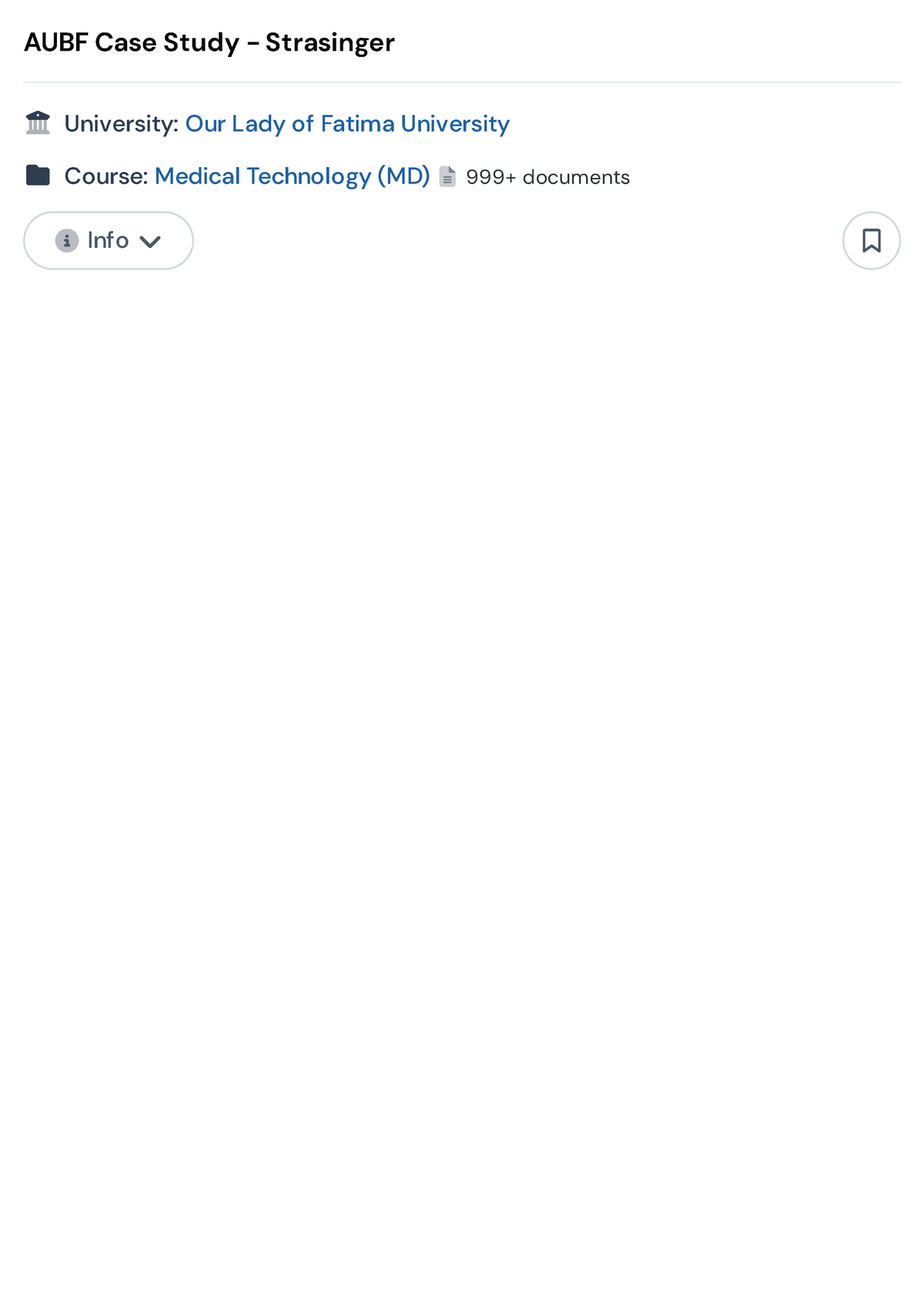This digital image, likely captured on a phone or computer, features a predominant white background. At the top, bold black text reads "AUBF CASE STUDY-Stratsinger." Below this, there is a visual element resembling a monument or building with the word "University" next to it, followed by a colon. In blue text, it states "Our Lady of Fatima University."

Underneath, there is a black icon resembling a file folder, with the label “Course:” in black text next to it. In blue text, it specifies "Medical Technology MD." Adjacent to this, a gray paper icon is displayed, indicating "999+ documents." At the bottom of the image, there is a clickable button for additional information, accompanied by a drop-down menu.